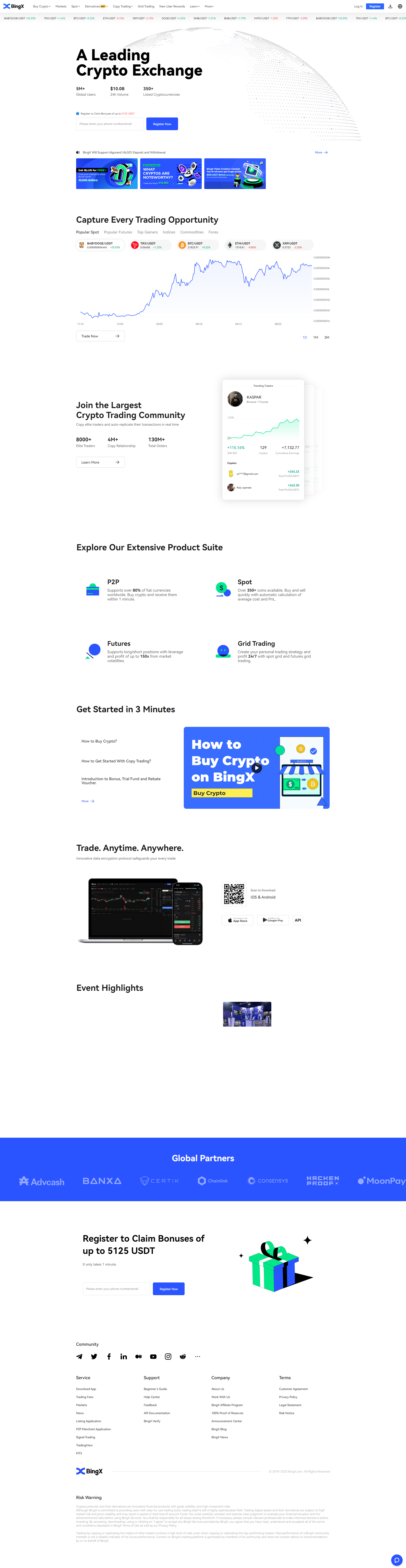This detailed and cleaned-up caption describes the layout and elements of a vertical image, most likely a screenshot from a cryptocurrency exchange website:

---

This vertical image appears to be from a cryptocurrency exchange website, ideal for viewing on a smart device. 

At the very top, the white background seamlessly blends with the screen, creating a cohesive look. In the upper-left corner, there's a blue "X" icon accompanied by the text "Bing X" in black. 

Navigational options are clearly listed, starting with "Buy Crypto," "Market," "Spot," "Deviations," and a highlighted yellow option labeled "Copy Trading." Other options include "Grid Trading," "New User Rewards," "Learn," and "More." 

On the upper right side, you can see buttons for "Login" and "Register" (the latter being in blue), a "Download" button, and a globe-like icon.

A light gray strip on the left side displays various trading icons and terminologies, showcasing numbers in both green and red along with black titles. The text "A Leading Crypto Exchange" is prominently displayed, providing an introduction to the platform. There's a registration field for users to enter their phone number and email.

The image also features blue information boxes about cryptocurrency, including a chart and various icons illustrating the platform's extensive product suite. Key points mentioned are the ability to get started in three minutes and the flexibility to trade anytime, anywhere. 

Additionally, there are event highlights and QR codes for iOS and Android downloads. At the bottom, the text "Global Partners" is mentioned along with an offer to "Register to Claim Bonuses of up to $5,125 USDT." The footer includes social media icons and more detailed information about the platform.

---